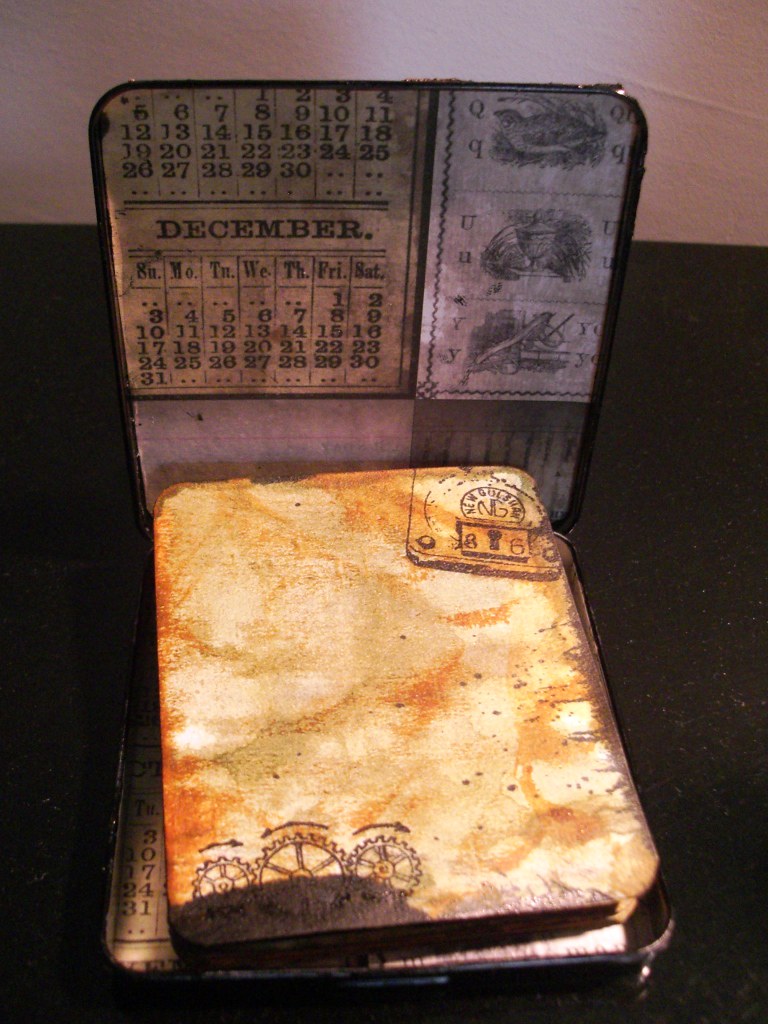The image depicts an old, rectangular metal tin, cracked open and placed on a dark, possibly black surface. The backdrop consists of stark white walls. The inside lid of the tin displays a printed calendar for December, featuring the days of the week from Sunday to Saturday. Below this are the days of the month. The calendar appears to be printed in an old style, on what looks like aged paper.

Inside the tin lies a discolored, tattered book that might have once been white but now shows a range of cream, beige, and yellowish-brown hues, suggesting it is very old. The book features a series of stamps and ink marks, including a specific gear logo with arrows in one corner, leading to the speculation that it could be a manual for gear making. The overall setting of the tin and its contents is defined by their vintage and worn appearance, with details such as little stamps and the visible numbering adding to the sense of historical significance.